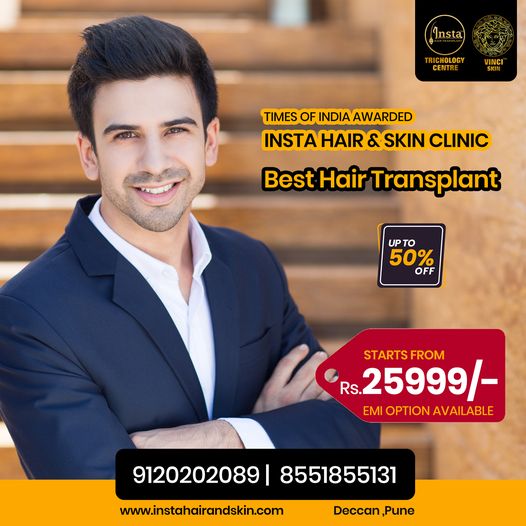This square advertisement poster showcases a man with brunette hair, dark eyebrows, dark eyes, and a slight beard and mustache. He is smiling, dressed in a dark navy suit with a white dress shirt underneath, and has his arms folded, presenting a confident and successful demeanor. The background appears to be brown, potentially resembling a door or shutters. In the top right corner, there are two logos: one for "Insta Trichology Center" and another with indistinct details, possibly "Vinci." The primary text, highlighted in yellow on a black background, reads: "Times of India awarded Insta Hair and Skin Clinic Best Hair Transplant." Below, there's a small graphic offering "Up to 50% Off" and a red price tag indicating "Starts from RS-25999. EMI option available." At the bottom, contact details are provided with two phone numbers: 9120-2020-2089 and 855-1855-131, followed by the website www.instahairandskin.com and the location "Deccan, Pune." The text colors vary between black, white, and yellow, making it visually striking.